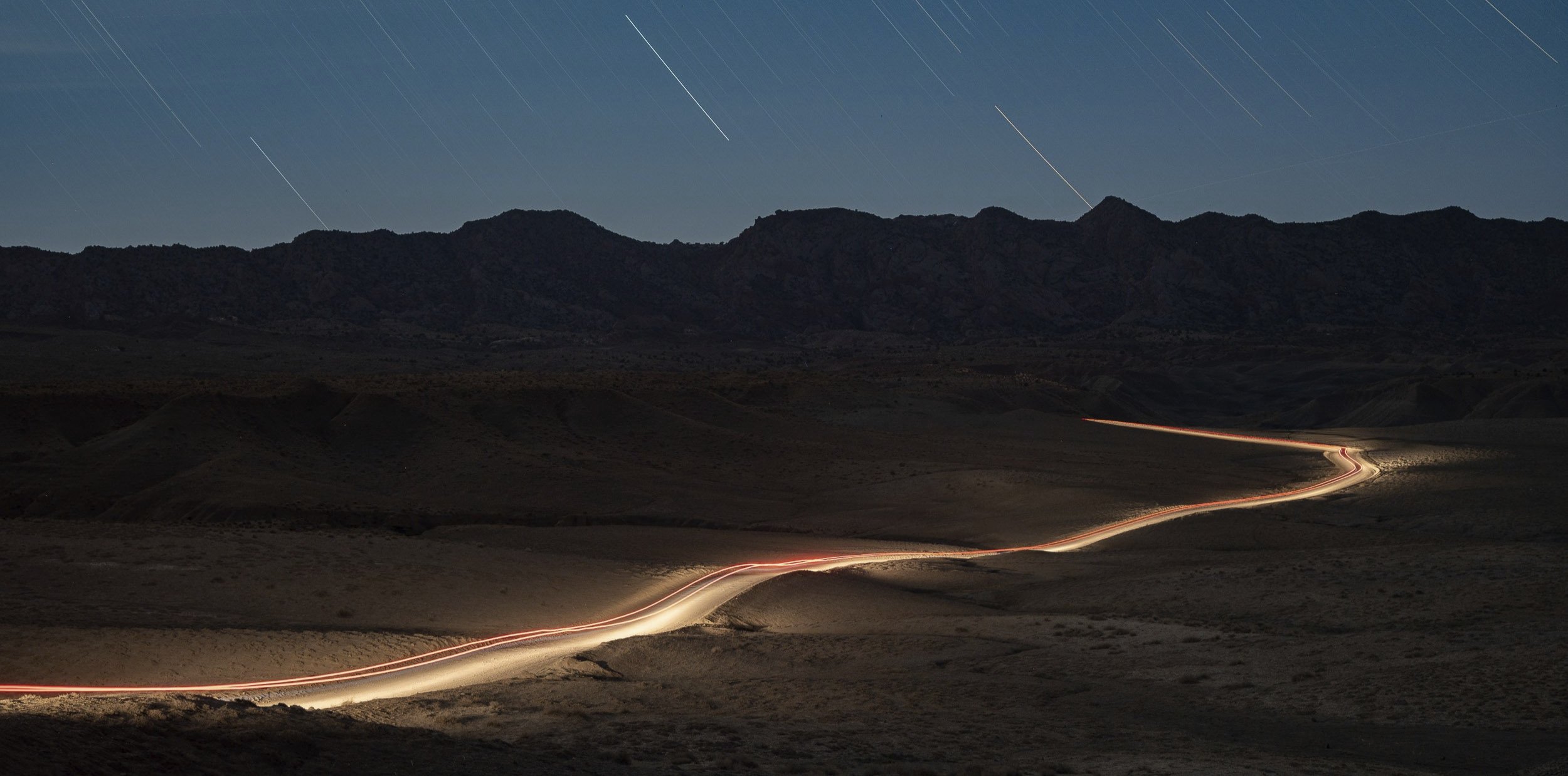The image is a stunning, enhanced color photograph of a desert landscape captured at dusk, characterized by a wide, horizontal orientation. The scene is most likely taken from an elevated viewpoint, possibly a drone, providing a sweeping view of the arid terrain. A narrow, winding road emerges from the bottom left corner, illuminated with a white glow, traversing the expanse of light brown sand. The road snakes its way up to the center-right portion of the image, where it makes a dramatic left turn before disappearing into a range of dark foothills.

The background features a mountain range that stretches across the entire width of the image, silhouetted against the darkening sky. The sky itself is a deep blue, indicative of the sun having just set. Adding to the ethereal quality of the image, a meteor shower with shooting stars appears throughout the upper part of the sky, creating little white streaks that further enhance the scene. The photograph's realism is accentuated with filters, subtly enhancing the natural elements to produce a visually captivating and cool depiction of a desert road at twilight.